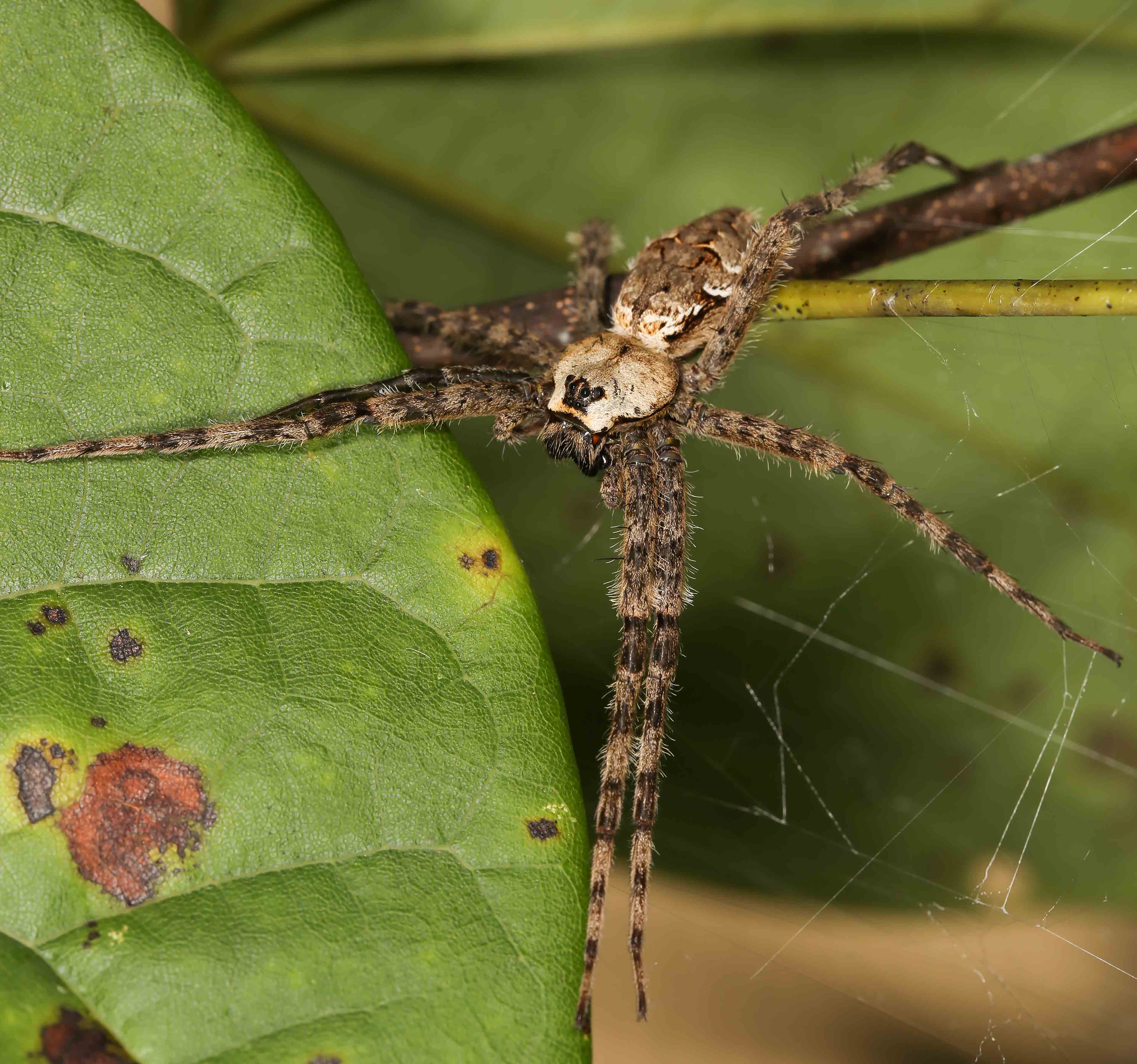This image features a large, hairy spider prominently positioned on the stem of a plant. The spider’s elongated, oval-shaped body comprises two distinct sections: a white head adorned with a small, crown-shaped black marking above its eyes, and a brown thorax with fine white lines. Its spindly legs, extending approximately three times the length of its body, display alternating cream and dark brown rings. The spider is partly situated on the stem while some legs stretch out onto nearby leaves, including a large, splotched leaf on the left side of the picture. Beneath the spider, a delicate, airy cobweb indicates recent activity, suggesting the spider is in the process of constructing its web.